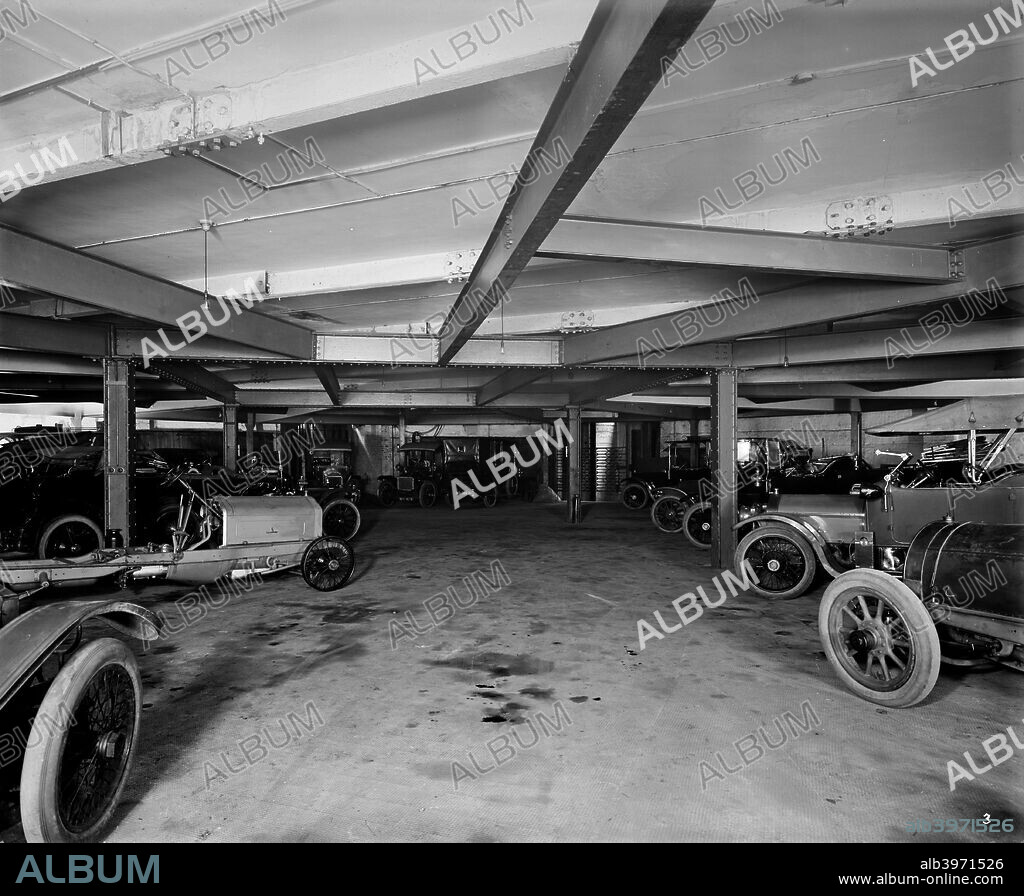The black and white photograph depicts a historic garage filled with vintage cars reminiscent of those from a hundred years ago. The image is dominated by shades of black, white, gray, and a dark bluish-gray tone. On the left side of the picture, there's an old car, while other similar cars are lined up in various parking stalls across the scene. The garage features a white ceiling with dark gray metal beams supporting it, and the ground appears slightly dirty with some dark gray patches. A watermark reading "album" is repeatedly stamped across the image in varying shades of white and gray. At the bottom of the photograph, a black bar displays the text "album" in a bluish-gray font on the left and "ALB3971526" followed by "www.album-online.com" on the right.